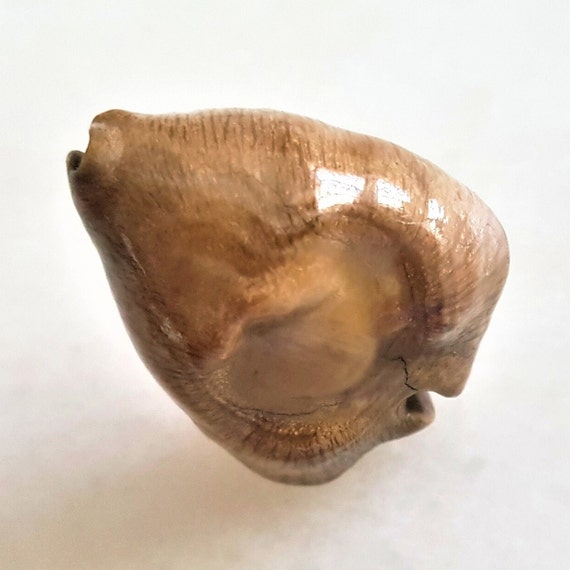This image depicts a shiny ocean seashell resting on a stark white surface that accentuates its contours. The shell is primarily light brown with a mix of darker browns, tans, yellows, blacks, and hints of gray, giving it a multi-colored appearance. Its shape is somewhat of a rounded triangle, nearly rectangular at certain angles, and it features two openings at either end, possibly serving as entrances or exits. The shell has a noticeable crack and a dent along one side. Its surface is highly reflective, capturing the light and enhancing its detailed textures and intricate patterns.